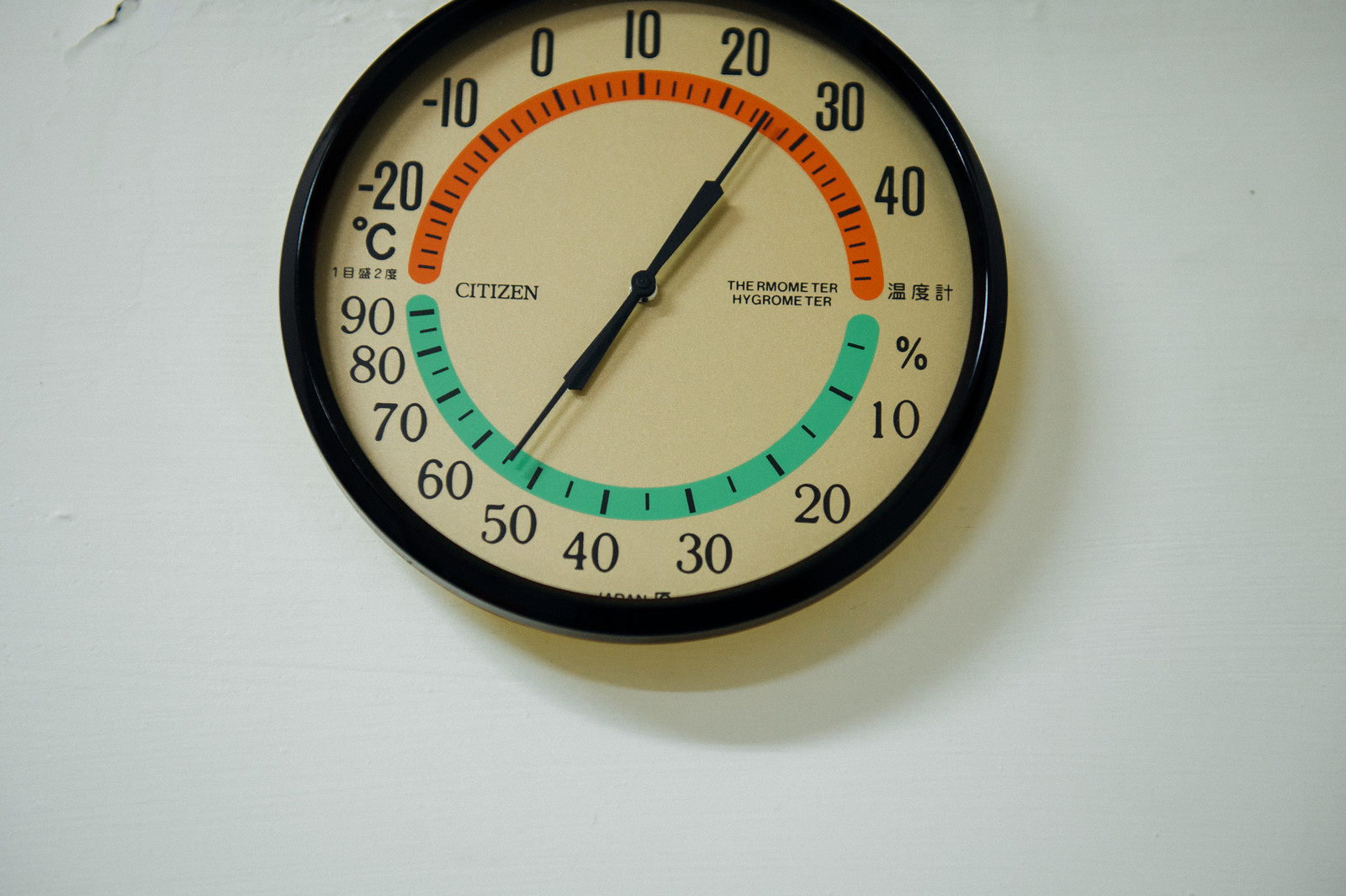The photograph showcases a round, black analog thermometer mounted on a white wall with noticeable dimpling. The wall's texture is accentuated by the round shadow cast by the thermometer. The thermometer's face, which is somewhat dingy with an off-white hue, prominently features black numbers and text. At the center, the brand name "Citizen" is written, followed by "Thermometer" and "Hygrometer", both of which include English and what appears to be Japanese or Chinese characters.

The thermometer measures temperatures in both Celsius and Fahrenheit. The Celsius scale, located at the top, ranges from -20 to 40, while the Fahrenheit scale at the bottom ranges from 10 to 90. An orange line with black dashes marks the upper section, and a robin's egg blue section with black dashes indicates the lower part. The overall design is both functional and aesthetically intriguing, blending precise measurement with a slightly aged appearance.